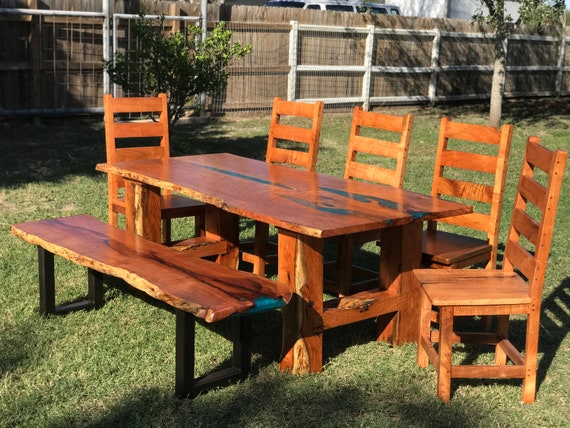This photograph captures a serene backyard scene bathed in bright daylight, evidenced by the lush, green grass and the sunlight illuminating the surroundings. Central to the image is a robust picnic table made of natural, brownish wood with a glossy, lacquered finish that accentuates its thick, heavy-duty legs and solid construction. The table, positioned diagonally in the center, is accompanied by a mix of seating: a bench with a black metal frame on the left and five wooden chairs—one at each end of the table and three along the back right side, all featuring slat backs and wooden seats. Despite the rustic charm of the setup, the table shows some rough edges, contrasting with the well-kept appearance of the chairs. The backdrop includes a seven to eight-foot tall wooden fence of medium-tone planks, with light-colored posts interspersed, and a mix of green foliage, including a small tree on the left and a gray tree trunk on the right. The scene is devoid of any food or decorations, suggesting the setup might be for an anticipated gathering or simply showcasing the furniture.